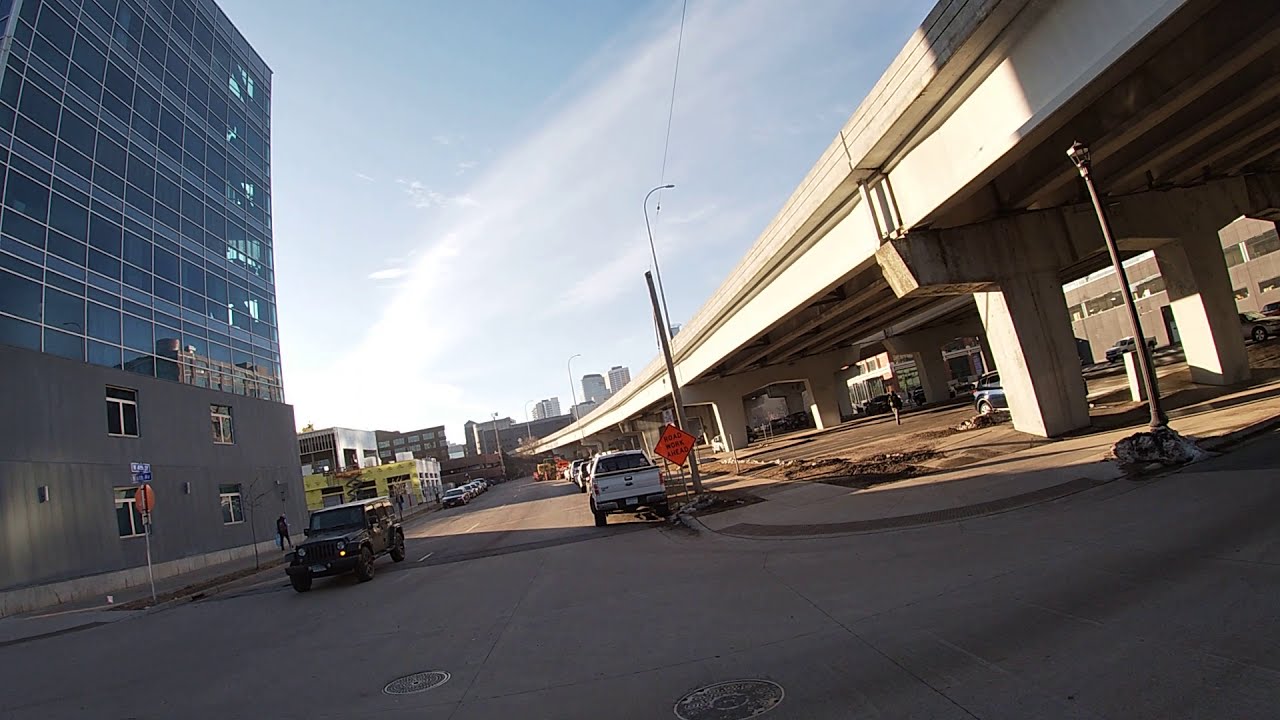This full-color landscape photograph captures a partly cloudy urban setting near a city, characterized by infrastructural elements and ongoing construction. Taken from the perspective of a person standing on the sidewalk, the image shows a street with two lanes in each direction. A dark-colored Jeep is preparing to turn toward the bottom left corner, while a white pickup truck is parked on the right side of the street. Further down, numerous cars line both sides of the road.

Dominating the right side of the photograph is a bridge overpass with concrete columns, curving from the top right toward the center, leading into the horizon. A construction sign indicates road work ahead, underscoring the development in this area. On the left, a multi-story building with a glass front above the second story stands prominently, possibly a parking deck or an almost-completed construction project. This building shares the vicinity with another building under construction visible in the distance.

High-rise buildings form the far background, adding to the urban atmosphere. A pedestrian is seen walking away from the screen, and blue street signs are visible near a stop sign on the left. The overall scene embodies a photographic realism style, capturing the intricate details and dynamic composition of an evolving cityscape.